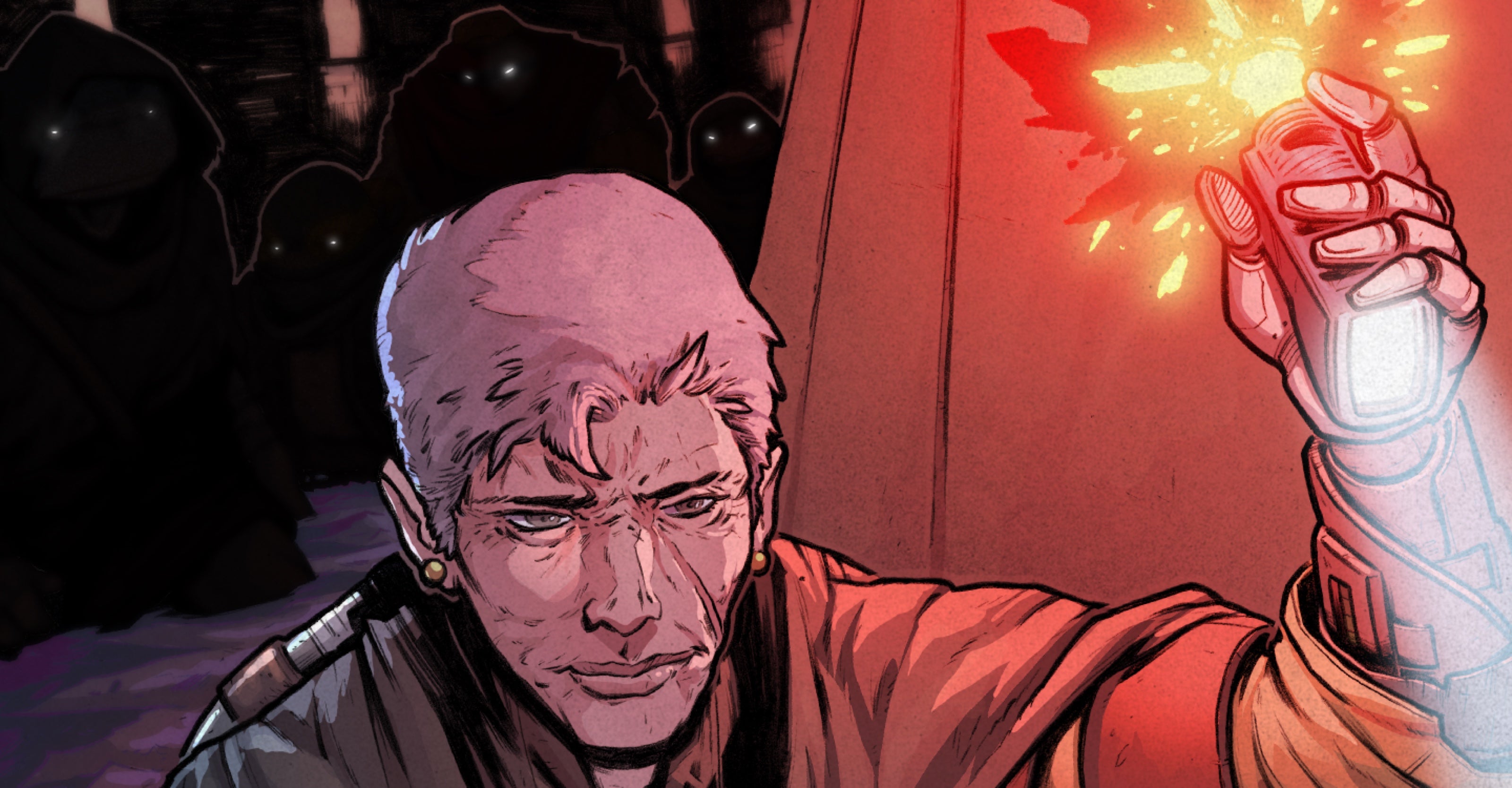The cel-shaded digital art piece depicts an older, androgynous individual, possibly in their 60s or 70s, with short, white hair and wearing a functional or military-style uniform. This person, sporting earrings in both ears, holds a forward-facing flashlight in their left hand. Intriguingly, the flashlight's back end emits sparks resembling a small explosion or fire, adding to the surreal atmosphere. The person features a determined expression and stands against a wall, suggesting they're entering a passageway or doorway. In the background, ominous cloaked figures with multiple glowing eyes add an eerie, unsettling vibe, emphasizing the likely sci-fi setting where something ominous seems to be unfolding.